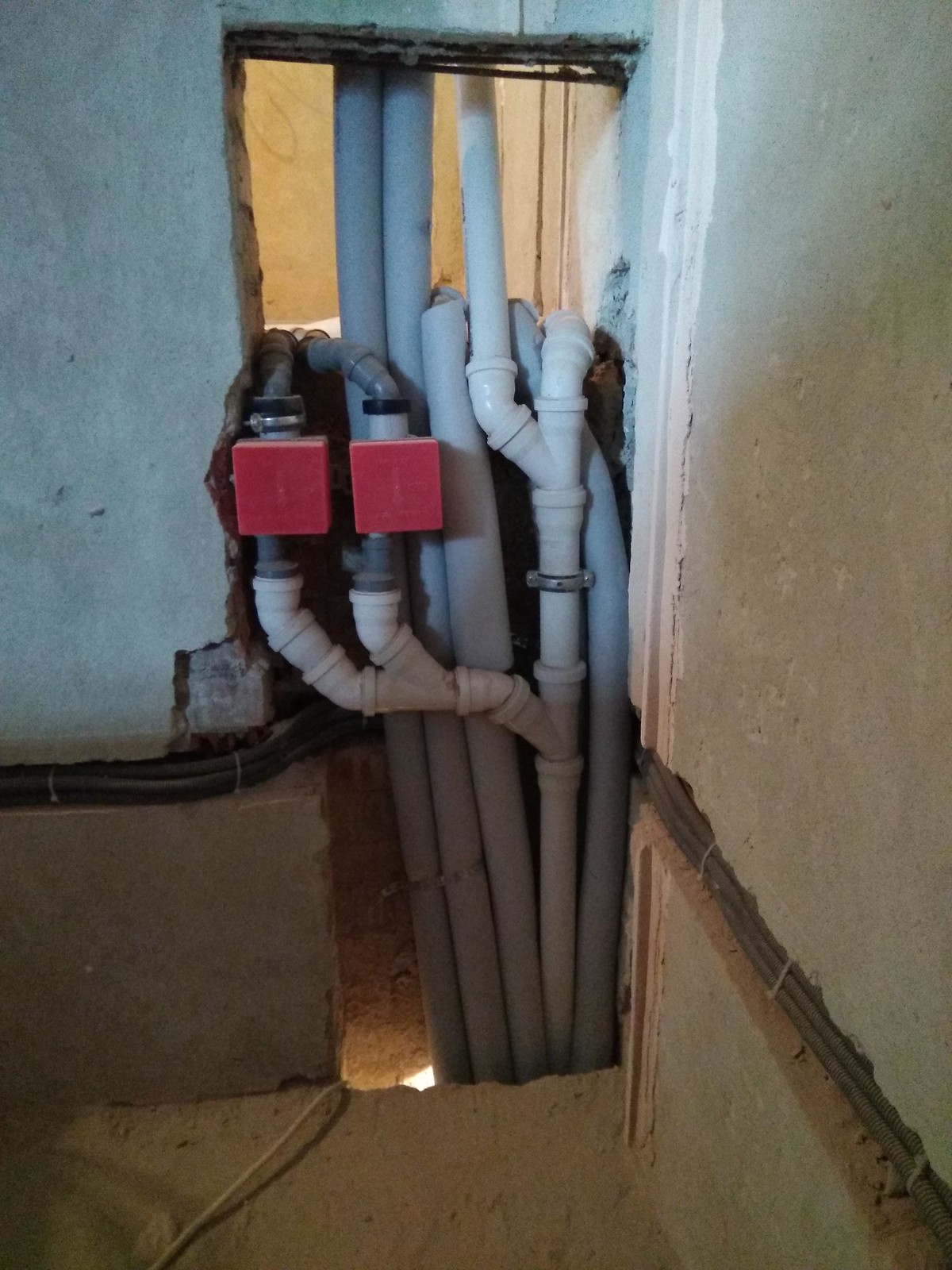The image depicts a basement-like area with a complex array of plumbing and cabling against a cut-out section of the wall. On the left, the wall protrudes about two inches before being abruptly cut away, revealing white water pipes that extend both vertically and horizontally. These pipes feature numerous connections, with some linking to two prominent red boxes positioned centrally in the image. From these red boxes, gray tubes ascend while white tubes plunge downward and then converge into a larger white pipe. Additional gray tubing accompanies the main structure, with one gray pipe on the right and three on the left; the leftmost pipes extend out of the frame, while the remaining tubes curve back upwards.

The wall itself is light blue for the upper two-thirds, transitioning to brown near the dirt-covered floor. Visible at the top is a thin line of uncut wall just before the damage starts. Running horizontally from the left, black tubing stretches out and intrudes into the image by about a third. A grayish wall moves toward the camera, adding to the scene's depth. The chipped and broken wall signifies recent alterations, and light filters through from both the ceiling and ground, highlighting the rough, white concrete floor scattered with dirt. In the foreground, a channel houses thick black cables tied together with zip ties, aligning parallel to the main pipes and creating an intricate network of utility conduits throughout the space.